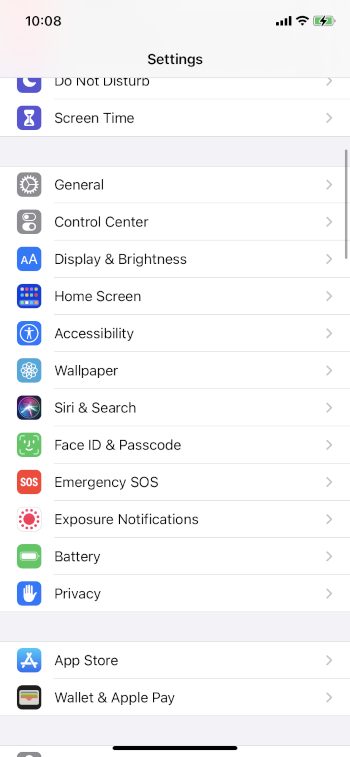The image depicts a screenshot of a mobile phone settings menu. On the left-hand side of the screen, the time is displayed as 10:08. In the middle, the word "Settings" appears in black lettering with a capital "S." To the right, there are icons indicating the signal strength, Wi-Fi connectivity, and battery status. The battery icon is green and features a lightning bolt, suggesting that the phone is currently charging.

The settings menu itself is organized into several sections. The first section includes a thumbnail image, possibly an avatar or app icon. Under this image, the first option listed is "Do Not Disturb." Following this, the menu options are as follows: 

- "Screen Time"
- "General"
- "Control Center"
- "Display & Brightness"
- "Home Screen"
- "Accessibility"
- "Wallpaper"
- "Siri & Search"
- "Face ID & Passcode"
- "Emergency SOS"
- "Exposure Notifications" (notably with capitalized "E" and "N")
- "Battery"
- "Privacy"

A thick gray bar visually separates the next section, which includes:

- "App Store"
- "Wallet & Apple Pay"

Another thick gray bar follows, with a small, half-width underline in gray at the bottom of the screen. The menu is well-organized, with each setting clearly listed in a clean and straightforward layout.